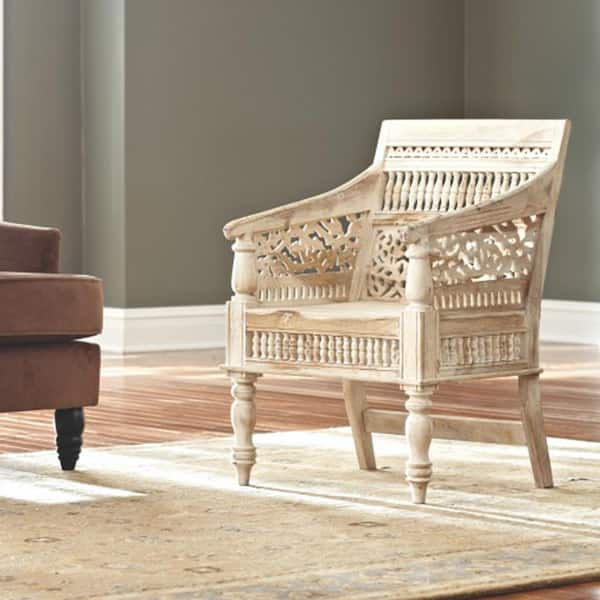The photograph captures an indoor setting featuring two distinctive chairs positioned on a cream-colored rug, which itself is placed on a brown wooden floor. To the center right of the image is a white wooden chair, notable for its simple design and white spindles, and it features a small white cushion for added comfort. To the left is a more modern chair, possibly a sofa chair, which appears to be primarily fabric with wooden feet and displays colors ranging from purple to beige. The room is characterized by brownish-gray or green walls with bright white trim along the bottom. The walls are relatively bare, reinforcing the minimalist aesthetic of the space. The overall setting appears minimalistic, with the two chairs as the focal points, facing each other as if awaiting occupants. There is no text or additional objects in the room to divert attention from the chairs and the rug beneath them.